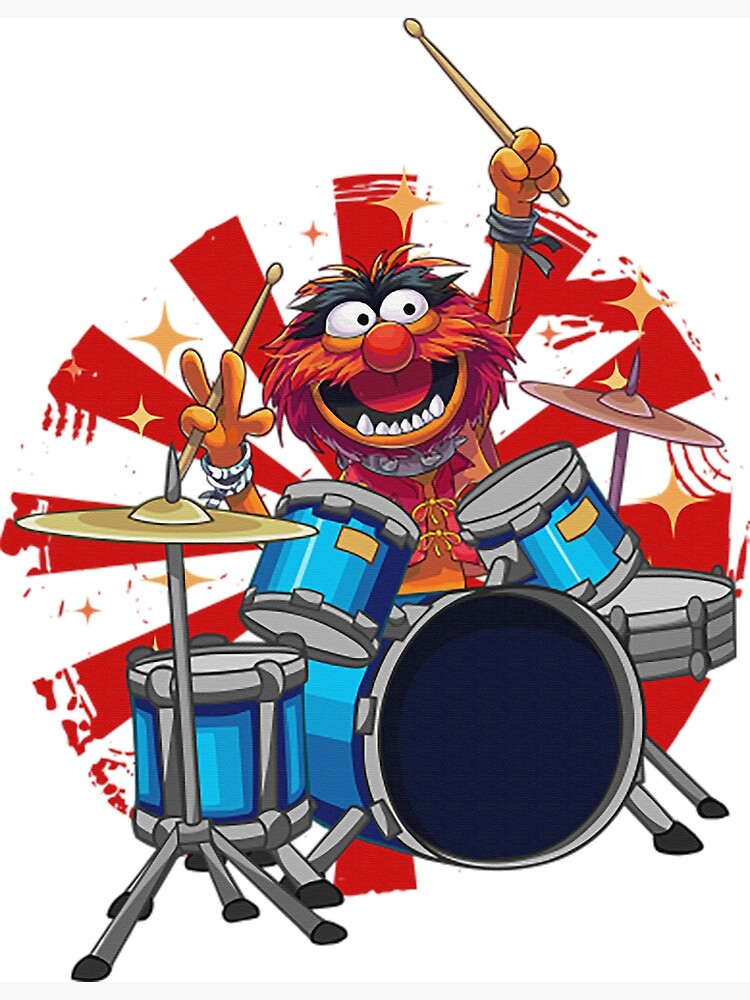This digital artwork features Animal, the exuberant drummer from the Muppets, sitting energetically behind his drum set. The drum set, prominently blue with metallic finishes, includes a large bass drum, two toms slanted towards Animal, a snare drum on the far right, and two cymbals—one on a stand to the left and another above the snare drum. Animal holds two drumsticks, his left hand (visible on the right) raised high, and his right hand (seen on the left) is held lower. He is clad in a spiked collar, a red vest, and matching black wristbands on both wrists. The background explodes with dynamic red and white sunburst patterns interspersed with golden stars, giving the scene an electrifying and vibrant energy. Animal's big, gleeful smile, wide eyes, and the visible teeth add to the lively and spirited atmosphere, making him look as if he's caught in an exhilarating moment of drumming. The entire scene is set against a clean, white backdrop that enhances the vivid colors and dynamic composition.